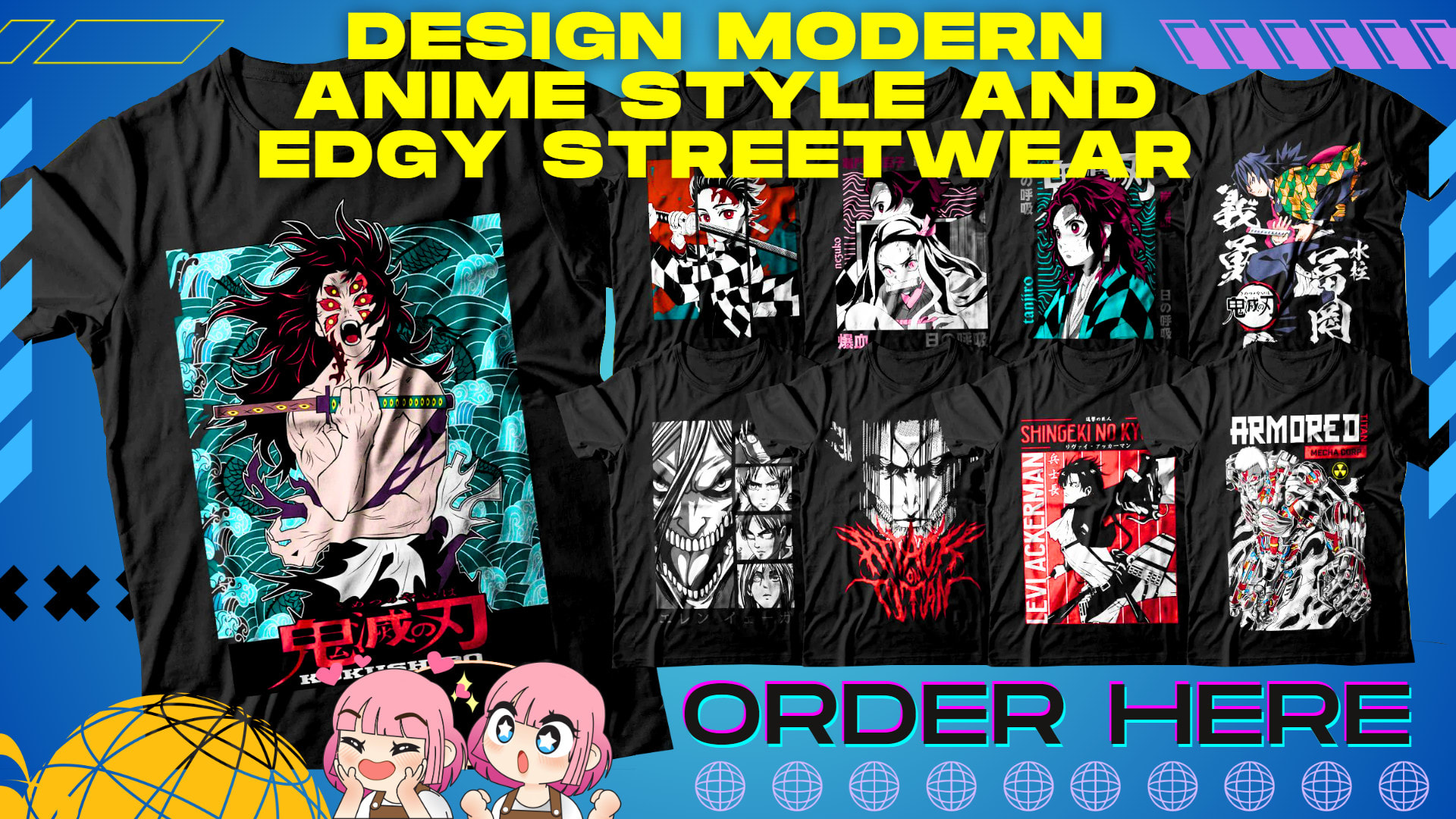This ad poster promotes a variety of graphic anime t-shirts, featuring bold designs that blend modern anime style with edgy streetwear. The background is primarily blue with hints of plum and light purple. At the top, in striking yellow text, it reads "Design Modern Anime Style and Edgy Streetwear." Below this, nine black t-shirts are displayed, each showcasing unique and edgy anime characters, some wielding knives or swords, some with creepy, wild faces, and decorated with Japanese text that suggests popular anime series like "Attack on Titan," "Demon Slayer," and "Street Fighter."

At the bottom left of the poster, two animated girls with pink hair and hearts around their faces capture attention. One girl has her hands over her cheeks, her mouth open in a surprised "ah" expression. The other girl exudes excitement, her eyes sparkling with stars and her mouth agape. On the bottom right of the poster, the call to action "order here" directs viewers on how to purchase the showcased t-shirts.